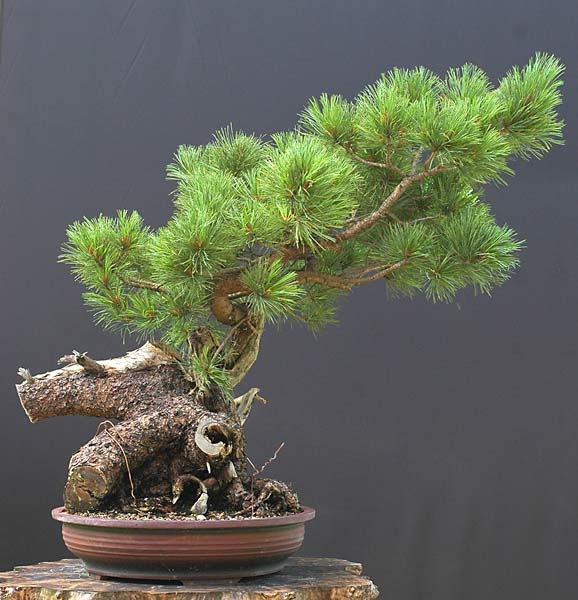In the image, a bonsai tree is positioned on the left side, placed within a short, wide, reddish-brown circular pot. The pot rests on a wooden platform that displays a jagged, circular shape transitioning through dark to medium brown hues. The bonsai tree, resembling a pine tree, features a truncated main stem with several cut branches, allowing a single prominent shoot to bloom. The tree's needle-like green leaves are plentiful and arranged in a manner that forms a floral shape. Brown seeds are visible where the leaves sprout from the branches. The background of the image is a flat, uninterrupted grey, providing a stark contrast that highlights the intricate details of the bonsai tree and its container.